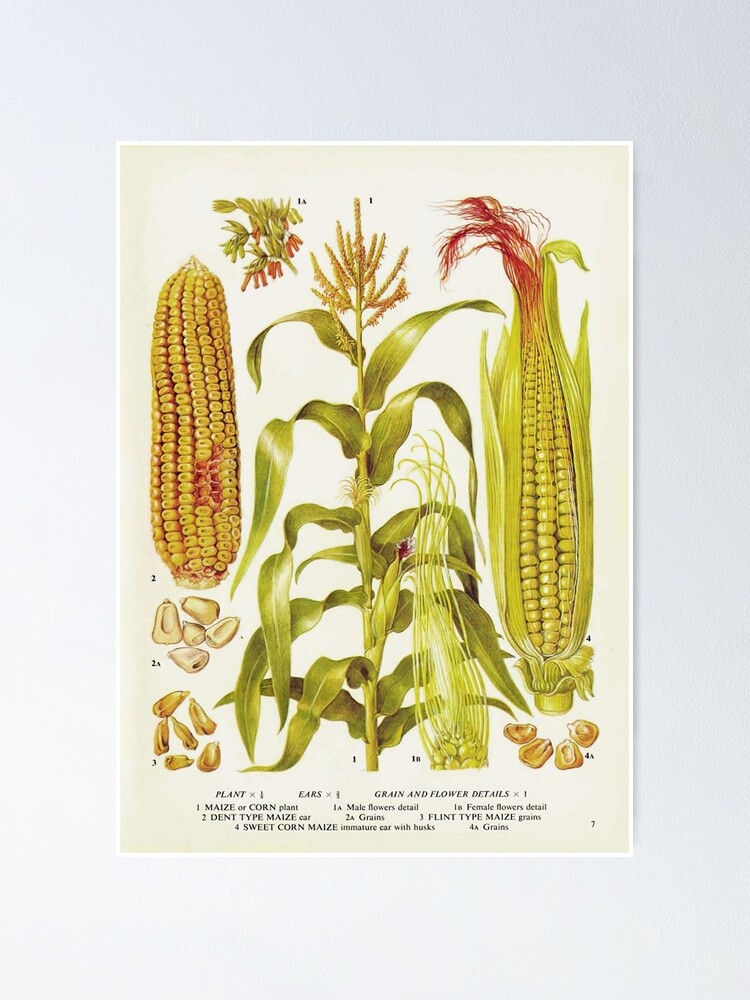This vertically-oriented poster with a sepia-toned white background provides an intricate depiction of various aspects of maize, also known as corn. On the left, a diagram labeled "2" features a huskless ear of dent-type maize, revealing neat rows of yellow kernels, some of which are labeled "2A" and "3" to denote different sections. Adjacent to this, you can see a collection of larger, detached kernels beneath the cob, suggesting stages of growth or varieties.

Centrally positioned is an illustrative maize (corn) plant, standing tall and robust with lush green leaves and a prominent tassel at the top indicating male flowers. The detailed rendering includes intricate green foliage, accompanied by delicate corn silk extending alongside. This segment is labeled as "maize or corn plant," highlighting the plant's structural and flowering details.

On the right side, an ear of immature sweet corn remains ensconced in its husk, prominently labeled "4." The husk reveals the distinctive reddish corn silk at the top, curling artistically, indicating the ear’s developmental stage. In addition, neat rows of kernels peek out from the husk, still attached to the cob, providing a contrast to the earlier fully exposed dent-type maize.

At the bottom, the poster includes a legend with comprehensive labels and descriptions for each corn type and part illustrated, including details about plant growth, grain types, and other horticultural specifics. The meticulous arrangement and labeling of elements suggest an educational or historical purpose, blending botanical art with informative content.